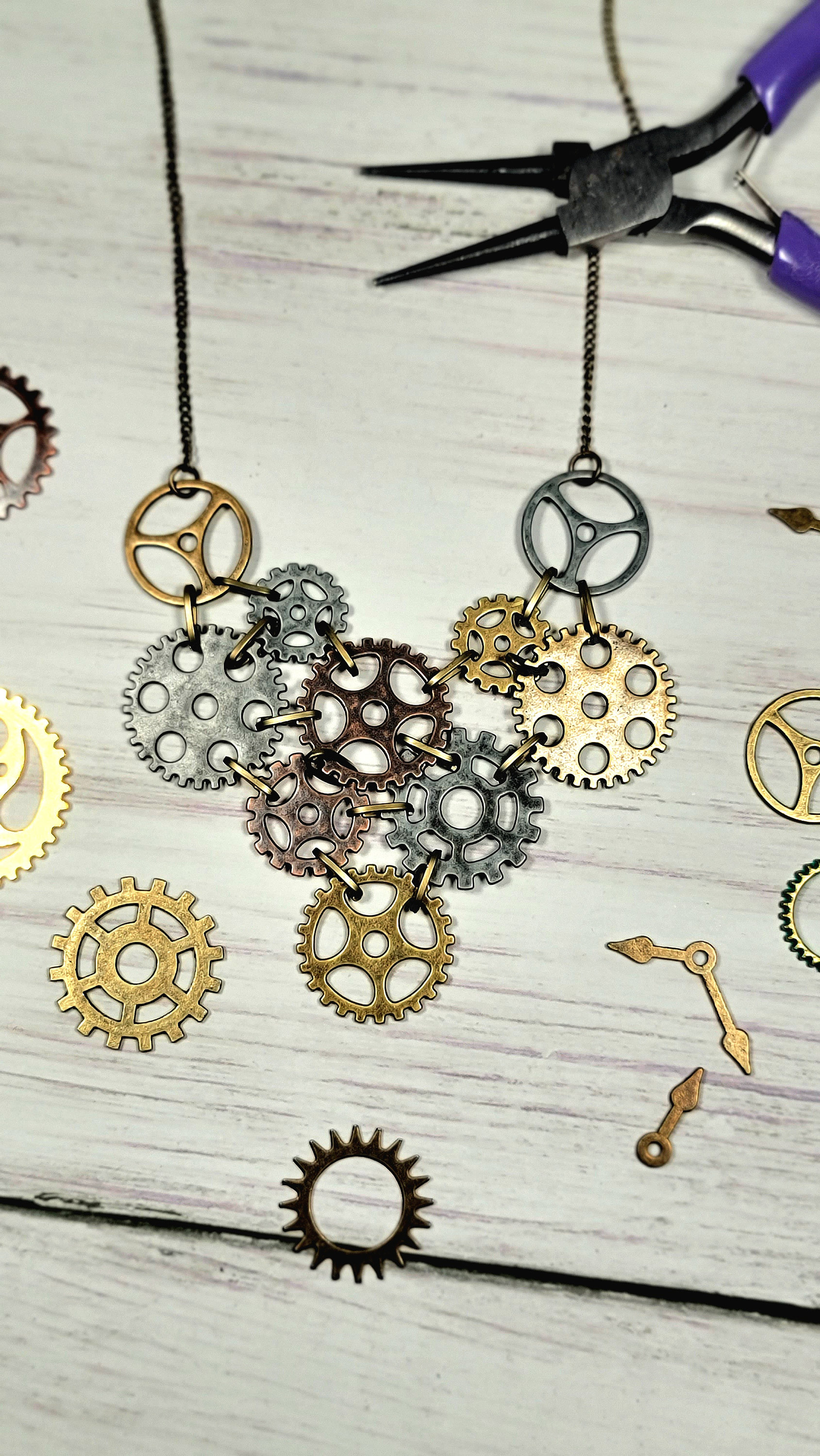This overhead photo captures a collection of metallic clockwork gears, intricately arranged on a wooden table. The gears, in shades of gold, bronze, and silver, are partially interlocked and strung together with dark metal rings, suggesting they are being transformed into a piece of jewelry, specifically a necklace. Scattered around are about a dozen gears, meticulously connected, with a dark-colored chain threading through them. In the top right corner, a metallic tool resembling wire cutters can be seen, hinting at the ongoing nature of this creative art project.